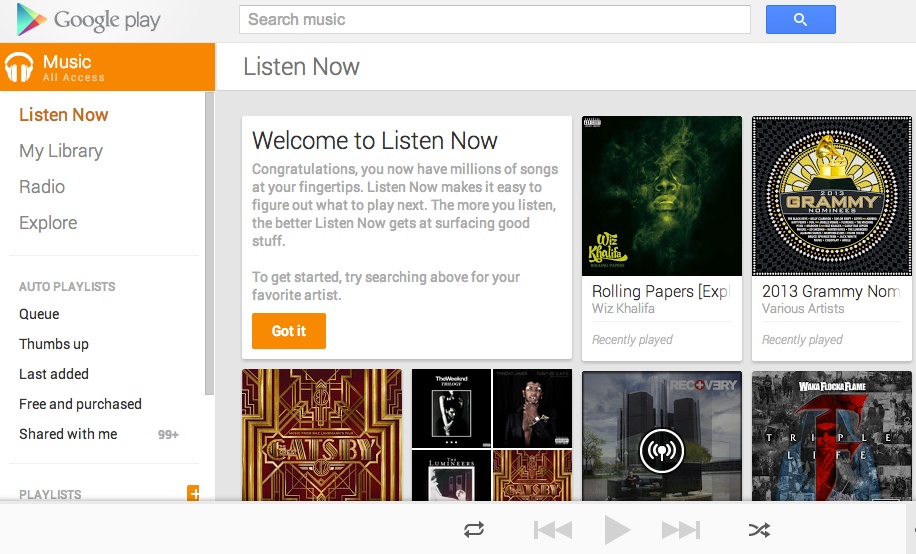The image is a screenshot of the Google Play Music interface on a computer. In the upper left corner, there is a colorful triangular logo with the words "Google Play" next to it. Adjacent to this is a search bar labeled "Search music," accompanied by a magnifying glass icon inside a blue rectangle.

Below the Google Play logo, the "Music" section is highlighted in an orange rectangle, reading "Music, All Access." Directly beneath this, there is another orange text, "Listen Now." Further down, the interface lists various sections such as "My Library," "Radio," "Explore," and "Auto Playlists." Subcategories like "Queue," "Thumbs Up," "Last Added," "Free and Purchased," and "Shared with Me" are also visible.

Near the top, under the search bar, the primary heading reads "Listen Now." Under this heading are several boxes representing different music options. In the top-left box, it welcomes the user with the text "Welcome to Listen Now," explaining they have access to millions of songs, followed by an orange "Got it" button.

To the right of this welcome box, there is a square featuring a dark, eerie image of an artist's face against a black background, labeled "Wiz Khalifa, Rolling Papers," with "Recently Played" beneath it. Adjacent to this is a circular badge showcasing the 2013 Grammy nominee, featuring a gold statue and captioned "2013 Grammy Nominee, Various Artists, Recently Played."

At the bottom of the screenshot, four additional squares display images of other artists and music tracks, though their titles are not visible.